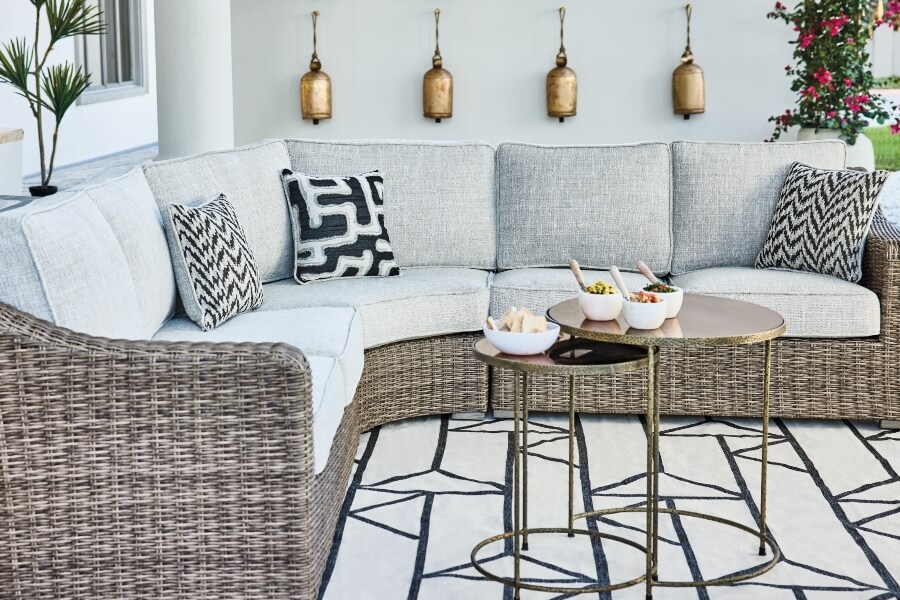This photograph captures a stunning outdoor living area that exudes the charm and sophistication of an indoor living room. The space features an L-shaped sectional couch made of an elegant wicker material, providing a robust yet chic foundation. Adorned with plush light gray cushions and stylish black and white throw pillows, the couch showcases a blend of comfort and contemporary design. 

The seating arrangement is accentuated by two round nesting coffee tables, each adorned with white bowls filled with decorative items and paired with white spoons. A white rug with a unique black line design, reminiscent of coat hangers, anchors the area, enhancing the inviting ambiance. Overhead, three lantern-style pendant lights add a touch of warmth while a potted fuchsia plant brings a pop of color and vibrancy to the scene.

To the left of the frame, a pathway suggests an easy connection to the outdoors, while the upper right corner reveals a glimpse of grass, confirming this exquisite setup is, in fact, part of an outdoor deck area. Behind the couch, the off-white gray walls and additional small plants contribute to the serene and airy atmosphere, making this an ideal spot for relaxation and entertainment in an open-air setting.